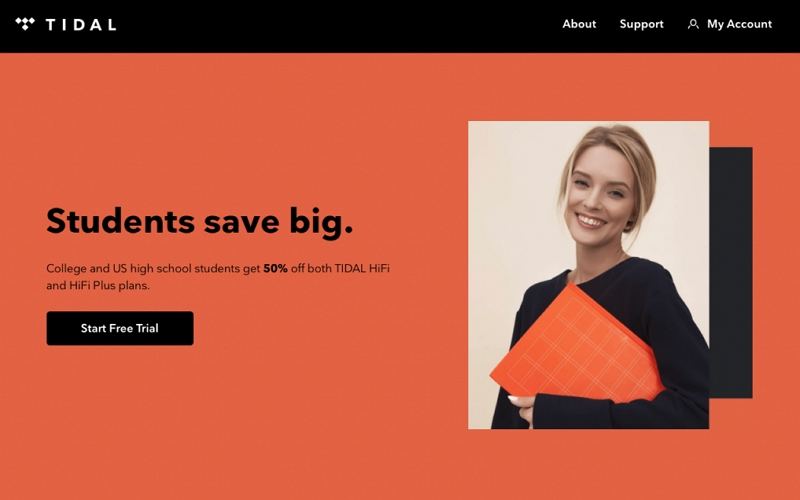The webpage features a modern design with distinct sections and vibrant colors. The top section has a black bezel, while the bottom half of the page showcases a burnt orange background. On the left side, there is a geometric arrangement of four squares forming an upside-down triangle. The prominent, bold white text reads "Title," referencing the music-identification service that helps users recognize songs.

On the right side, the webpage contains additional white tabs labeled "About" and "Support," along with an icon of a person represented by a circle for the head and two lines for the body, denoting the "My Account" section.

Highlighted on the left side with bold black text against a burnt orange background, it states, "Students Save Big." Following this, the text explains in regular black font, "College and US high school students get," with "50% Off" in bold black, for both "Title Hi-Fi and Hi-Fi Plus plans."

In the center is a black rectangle with white text that invites users to "Start Free Trial."

To the right, there is an off-white rectangular section featuring a light-skinned woman with short blonde hair, possibly tied in a ponytail. She is dressed in a long-sleeve dress shirt and holds an orange binder with muted white bands. Her fingernails appear to be painted white, and she smiles warmly at the camera. This off-white rectangle creates a shadow effect with an adjacent smaller black rectangle overlapping it slightly, adding depth to the page's layout.